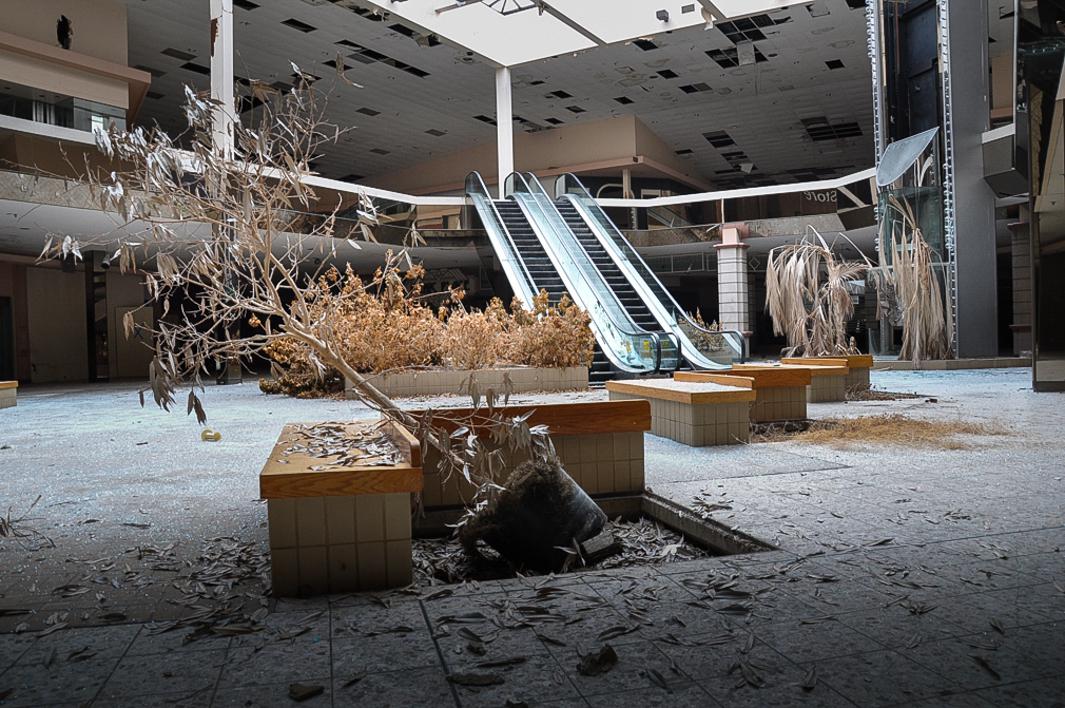This photograph depicts a dilapidated and abandoned indoor shopping mall, reminiscent of scenes from the 80s or 90s. The central court features two non-operational escalators ascending to the second floor, bathed in natural light from a damaged skylight above. The skylight itself shows significant disrepair, with several ceiling panels missing or dangling, exposing the underlying structure.

In the foreground, there is a sand-colored brick bench topped with wood, near which a potted tree lies tipped over, its lifeless, brown leaves scattered around. The area where the tree once stood is darker, adding to the desolate atmosphere. Throughout the mall, dead plants are prominent, including what appears to have been palm trees and shrubs now brown and dried out.

To the right-hand side, there is a non-functional elevator, further emphasizing the mall's abandonment. Small patches of grass or dead weeds have begun to grow between the tiles on the floor, and scattered debris is visible. The overall scene is bleak, characterized by muted tones of beige, gray, and white.